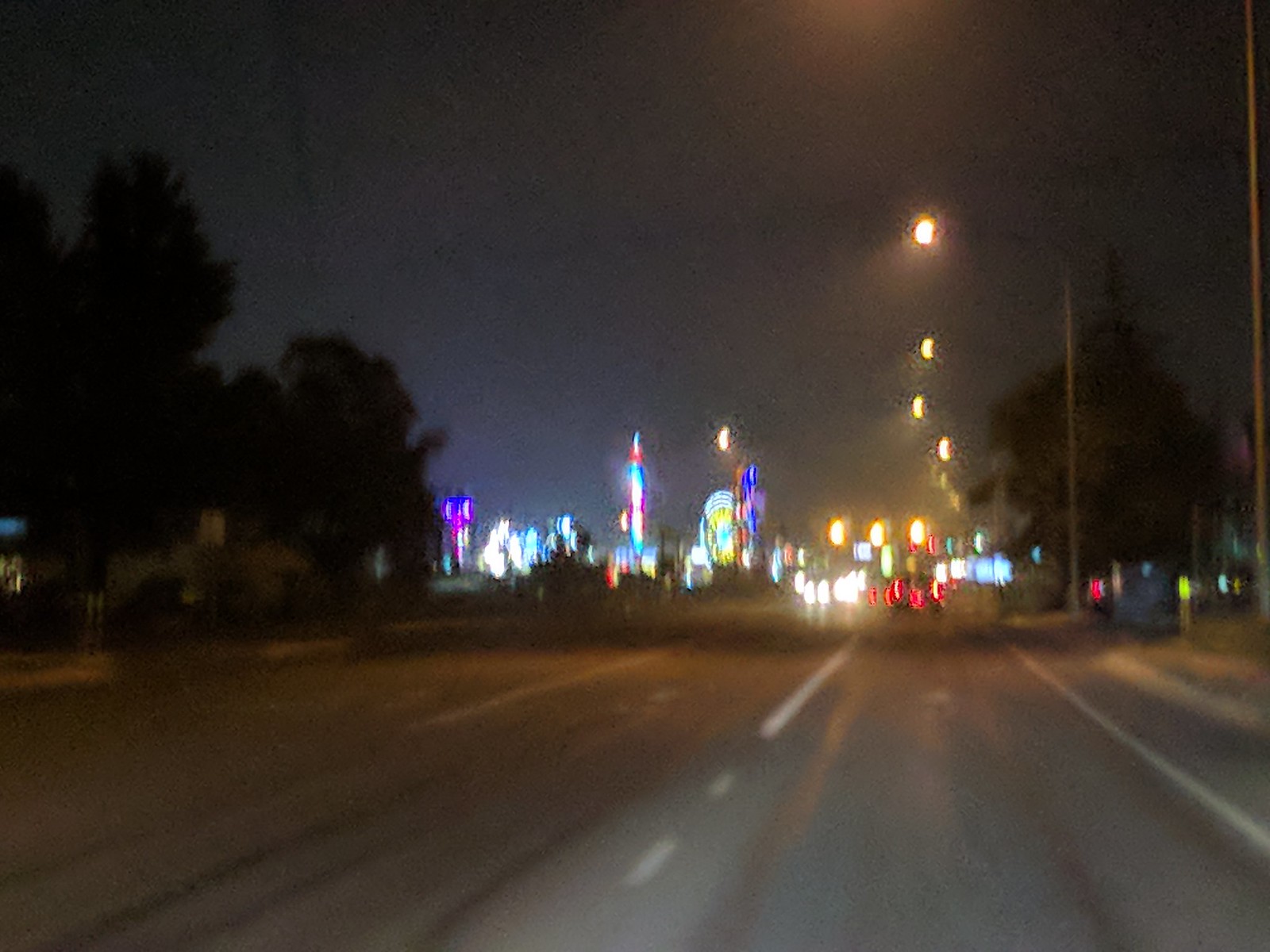This nighttime photograph, taken from within a moving vehicle, captures a blurred yet lively urban street scene. The camera angle places us in the middle of the road, which is marked with white stripes on the pavement. Tall streetlights glow with a yellow hue, casting a soft luminescence across the scene. Up ahead, brake lights from several cars illuminate the hazy night air, and a stoplight midway through its yellow signal hangs in the distance. Beyond, headlights of approaching vehicles frame a bustling downtown area on the horizon. A Ferris wheel and other brightly lit attractions suggest the presence of a carnival amidst the tall, illuminated urban buildings to the left.